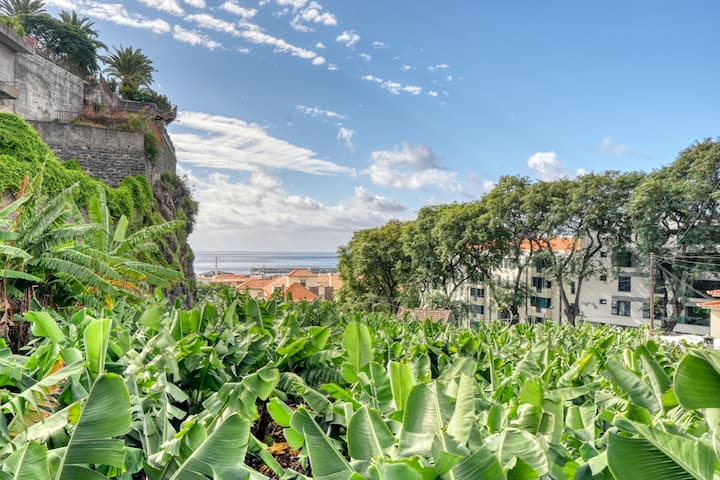In this vibrant, detailed photograph taken from a low vantage point amidst lush greenery, the foreground is filled with vibrant leaves, weeds, and an assortment of plants. The clear, sunny day showcases a bright blue sky dotted with a few clouds, adding depth without obstructing the sunlight. To the left of the image, a rocky cliff is visible, adorned with palm trees and some brick walls and balconies. On the right, there's a row of five tall trees, beyond which you can see white, three-story buildings, possibly apartment complexes. Peeking through the buildings, you can spot power lines against the backdrop of the bright blue sky. The center of the image offers a glimpse of a quaint town characterized by its terracotta-roofed Mediterranean-style houses, sitting serenely under the expansive sky. Beyond the town, the blue waters of the ocean stretch out to meet the horizon, creating a picturesque contrast with the lively greenery in the foreground.